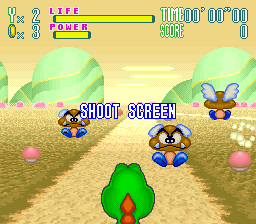This is a tiny, square screenshot of an old video game, likely from the 80s, featuring a cartoony and colorful scene. At the center of the image is the back of a green dragon-like dinosaur with orange or red triangular accents on his head and back, standing on a light golden dirt pathway that runs through the scene. The path is flanked by grassy areas and rounded, fantasy trees mirrored on both sides. In front of the dinosaur are three types of mushroom-shaped men with wings, reminiscent of creatures from Super Mario, poised as potential adversaries. In the center of the screen, the text "shoot screen" appears in white with a blue outline. The top of the screen shows life and power bars in yellow, labeled "Y X 2" and "X 3" respectively. To the right, it displays the time as 00:00:00 and the score as zero. The overall aesthetic of the scene combines elements of gold, green, pink, blue, and yellow, evoking a playful, fantasy land.